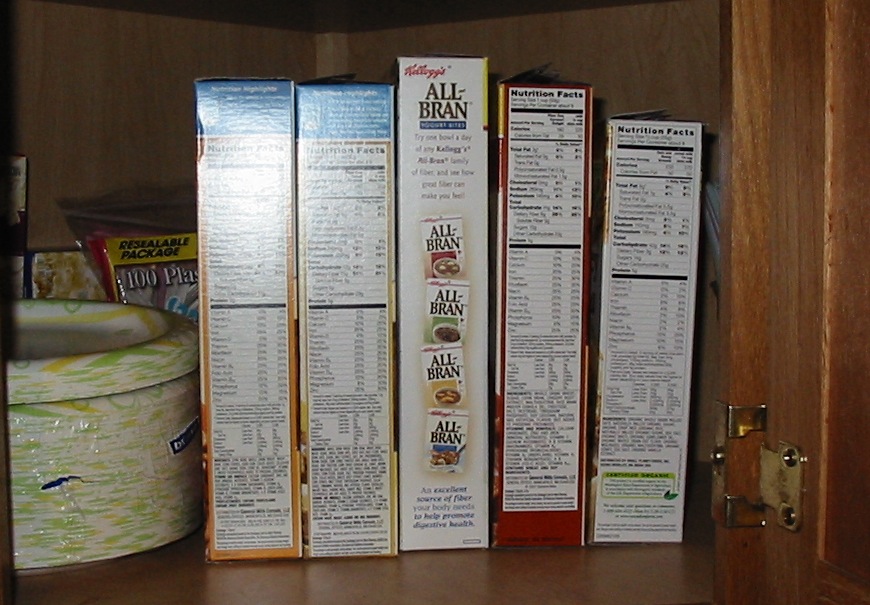This close-up photograph captures the interior of an open, chocolate and light brown wooden pantry. On the pantry shelf, there are five cereal boxes lined up, with the central box clearly displaying the label "Kellogg's All-Bran" in red and black text, along with small images illustrating the cereal variations in red, green, yellow, and blue. The labels of the other four boxes are predominantly showcasing nutritional information and are hard to identify. To the left of the cereal boxes, a tall stack of Dixie paper plates is partially unwrapped, featuring a white base with yellow and green stripes. Behind this stack, a plastic bag labeled "resealable package 100 PLA plastic" likely contains disposable spoons, forks, and knives. On the right side of the pantry, a brown door with gold hinges is visible.